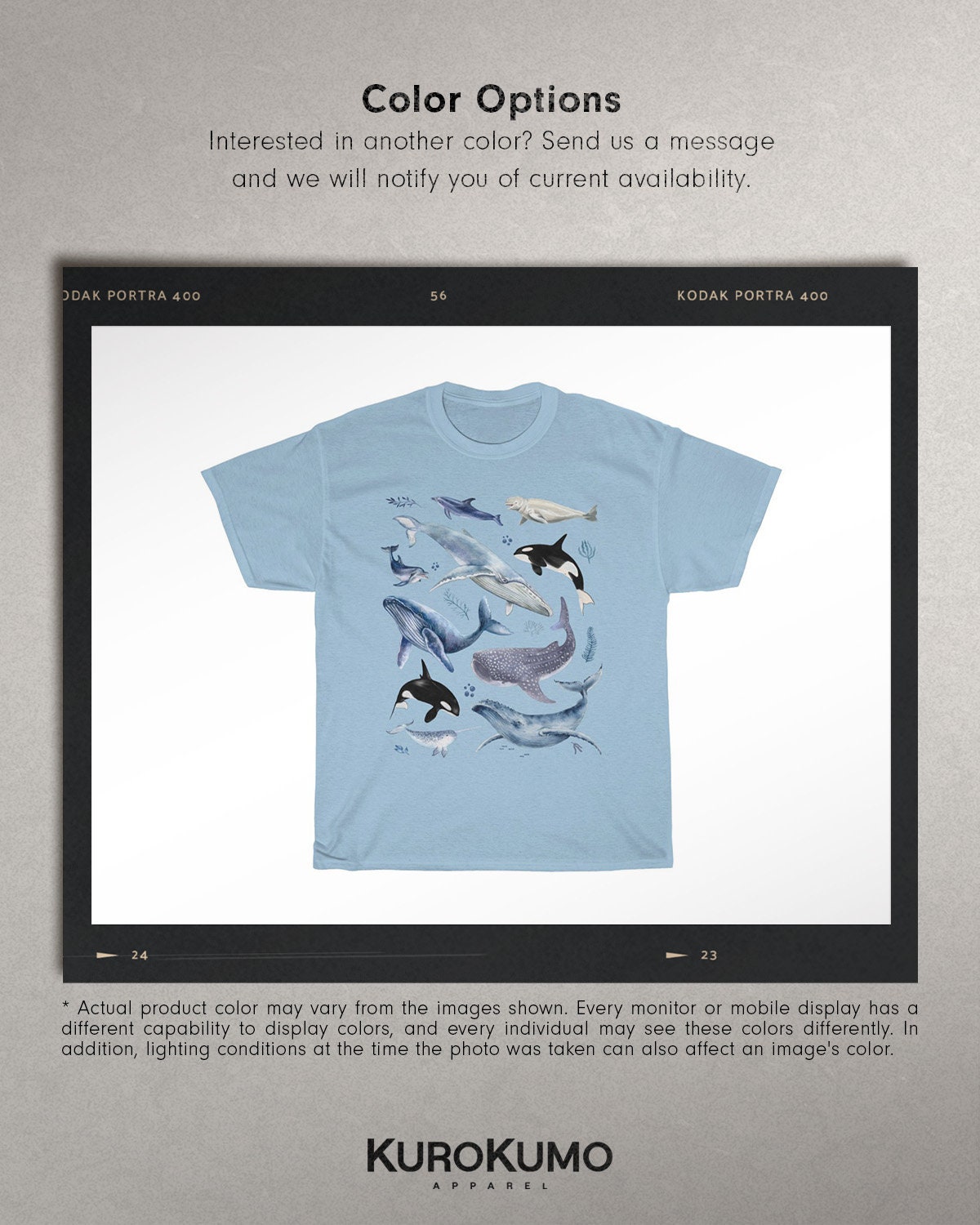The image appears to be a promotional photograph of a t-shirt from an apparel website, set against a white background. The t-shirt is light blue and features a lively and detailed print of various sea creatures, including orca whales, blue whales, humpback whales, beluga whales, and a dolphin in one corner. The design is further embellished with elements of marine vegetation like kelp.

The entire composition is framed in a style reminiscent of a Polaroid photograph, although it is not an actual Polaroid. Above the t-shirt, there is text that reads "Color Options" and offers an option to inquire about other colors: "Interested in other color? Send us a message and we'll notify you of current availability."

Additionally, there is an asterisk at the bottom of the text that leads to a disclaimer, explaining that the actual product color may vary from the images shown due to differences in monitor or mobile display capabilities and lighting conditions during photography.

At the bottom of the page, the name of the apparel company "Kuro Komo Apparel" is displayed.